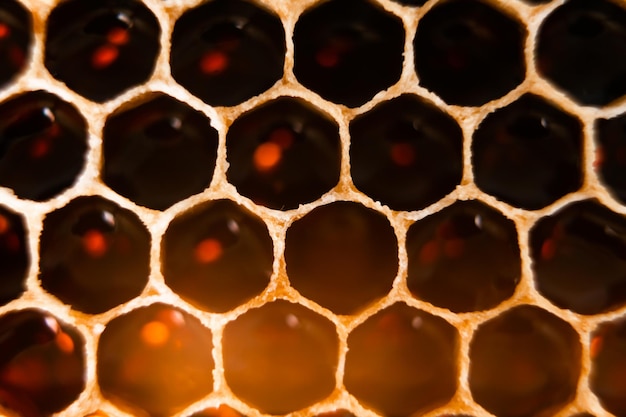This image presents a close-up view of a honeycomb-like structure, featuring rows of circular formations rather than hexagonal. The formations are outlined with a tan or beige border, while the interiors appear black, possibly filled with a dark liquid. There are four rows of these circular formations, with some partially cut off by the edges of the image. Scattered throughout the structure, especially in the upper left corner and lower sections, are red light splotches. Additionally, an orange glow permeates the bottom portion of the image, adding an interesting contrast. The overall effect is a harmonious blend of dark, tan, red, and orange hues, highlighting both the organic texture and the light interactions within the scene.